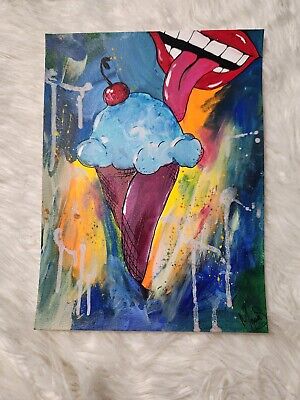The image is a photograph of a vibrant, stylized painting hanging on a textured, tan-white wall. The focal point of the painting is a blue ice cream cone with a cherry on top, adorned with little leaves. The cone itself is an unusual brownish-purple shade, featuring an enigmatic line halfway down. Above and to the right, a set of red lips with white teeth is depicted, with a large tongue extended to lick the ice cream. The background is predominantly blue but is enriched with dynamic splashes of orange, yellow, green, and white, giving the entire piece an abstract and colorful appearance. This detailed painting captures a whimsical and surreal moment, cleverly utilizing bold contrasts and vivid hues.